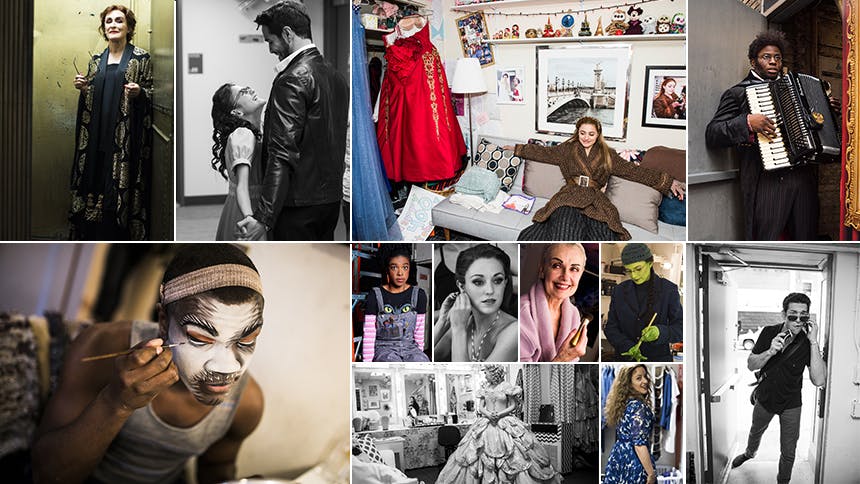This collage consists of six distinct images showcasing a variety of subjects and settings. 

In the top left, a woman wearing a black dress is seen standing in what appears to be an elevator, imbued with a sense of solitude. Adjacent to this on the right, a black-and-white photo captures a tall man in a leather jacket holding hands with a much shorter woman who looks up at him, both exhibiting a tender connection. Moving to the center-top, a woman dressed in a brown jacket sits on a richly appointed couch adorned with many pillows, surrounded by household clutter including photo frames and various trinkets. The top right image features a black man wearing glasses and a black jacket, playing an accordion, with a focused expression on his face.

On the bottom left, another photo shows an individual applying white makeup, perhaps for a stage performance or Halloween, their face partially transformed and attention absorbed in the intricacy of their task. The central bottom picture is a composite of six smaller photos predominantly featuring women in various dresses, with one figure in overalls, presenting a vibrant array of personas and styles. Finally, the bottom right image, also in black and white, depicts a man dressed in a black shirt and sunglasses walking through a doorway, exuding a sense of movement and purpose.

Altogether, this collage presents a rich tapestry of human experiences and interactions, from intimate moments and artistic pursuits to individual expressions and everyday life.